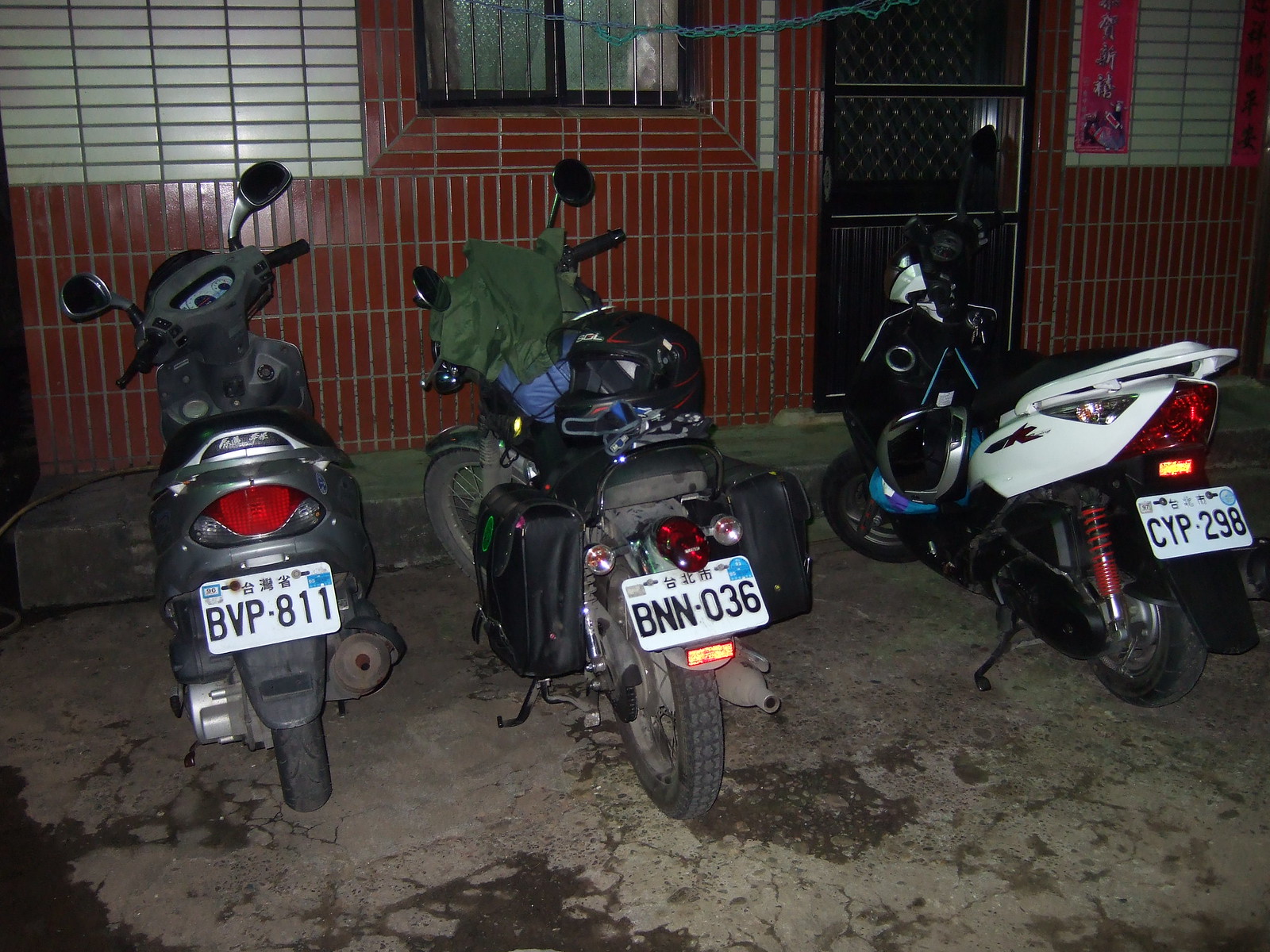The image displays three well-used motorcycles parked against a building on a dirty cement surface that appears stained or wet, possibly with oil. The building, constructed from shiny red and white tiles, has a black front door and two windows with bars. All three motorcycles face away from the camera towards the left. They each have white license plates featuring Asian characters in blue above black numbers and letters. Two of the motorcycles are black, while one has a white base. The motorcycles, with their rusted mufflers, seem to be of the scooter type and display signs of wear. There's some speculation about the building's purpose, whether it's a residence or a bar-like establishment, and a figure is faintly visible inside.